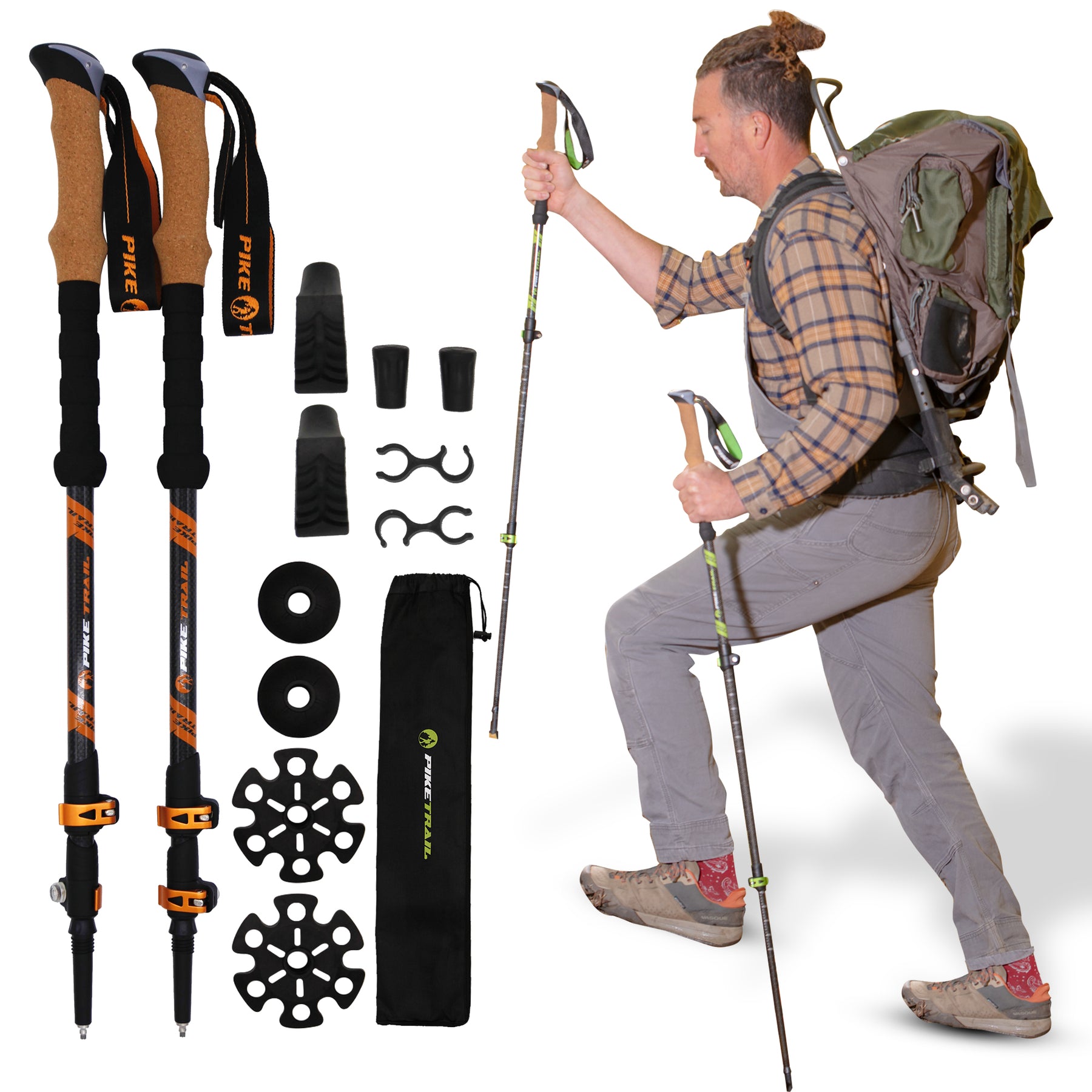The image showcases a comprehensive demonstration of hiking gear. On the left, there are hiking poles branded "Pike Trail," featuring ergonomic cork handles with black neoprene grips below. These poles are predominantly black with orange accents, including orange fasteners at the bottom. The display includes additional accessories such as coupling components to hold the poles together, gear storage solutions, and a carrying bag. To the right of the image, a man is demonstrating the use of the hiking poles. He has a dark hair bun and a mustache, wearing a plaid shirt in orange and light gray, gray pants, red socks, and brown sneakers. He also sports a gray and green backpack. The man is depicted in an active pose, one leg raised, effectively illustrating the poles' functionality.